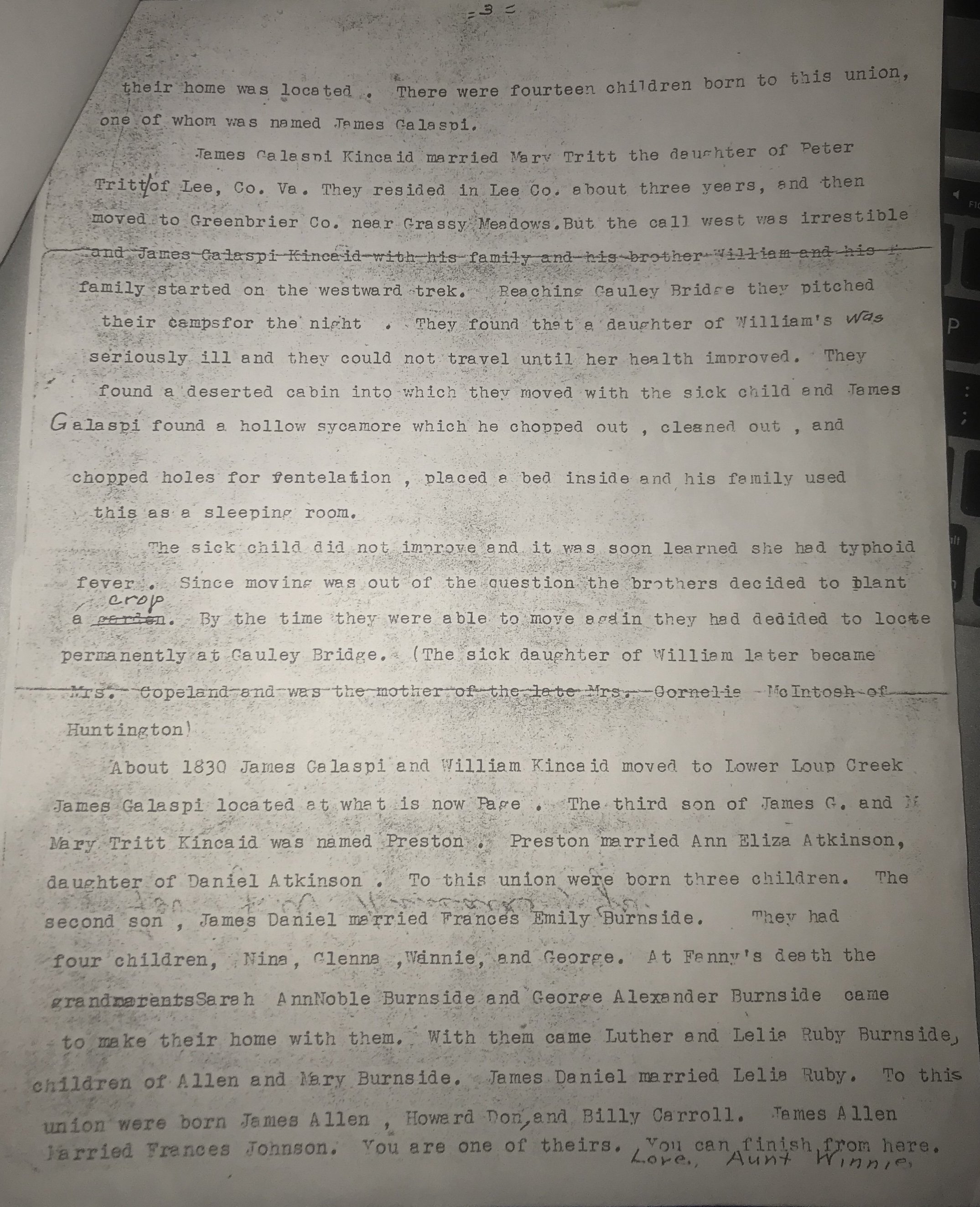This photograph captures what appears to be a photocopy of an old, typewritten document, characterized by a number of imperfections such as smudges and creases indicative of its age. The document, folded into thirds at some point, possesses significant horizontal creases, suggesting repeated handling. It also has a staple or paperclip in the upper left corner, attaching it to another partially visible, folded piece of paper.

In the upper right corner of the image, there's a glimpse of a laptop with black keys on a gray background. Additionally, there is a blank piece of folded paper found adjacent to it. The lighting of the photograph is somewhat dim, adding to the weathered appearance of the document.

Throughout the document, there are handwritten corrections made with a black pen, where certain words or sentences have been manually crossed out and revised. The typewritten text narrates the genealogical and migratory history of the Kincaid family. It starts with James Gillespie Kincaid who married Miss Marv Tritt, daughter of Peter Tritt of Lee, Virginia. The couple initially resided in Lee County for three years before relocating to Greenbrier County near Grassy Meadows. 

The story details a westward trek made by James Gillespie Kincaid, his family, and his brother William's family. During their journey, they camped at Galet Bridge, where William's daughter fell seriously ill with typhoid fever. The families settled temporarily in a deserted cabin and a hollow sycamore for shelter while they waited for her health to improve. By the time they were able to move, they decided to settle permanently in Galet Bridge. William's daughter eventually recovered and became Miss Copeland, mother of the late Miss Garnley Macintosh of Huntington.

Subsequent sections provide more genealogical details, noting that by 1830, James and William Kincaid had moved to the lower Loop Creek area, with James Gillespie settling in what is now Page. The document continues with details of marriages and births within the family, leading up to the present generation. In a closing note written in text rather than typed, there’s a personal touch: "Love, Aunt Winnie."

The combination of the historical narrative, the personal note, and the visible signs of age and use contributes to the document's rich, authentic character.